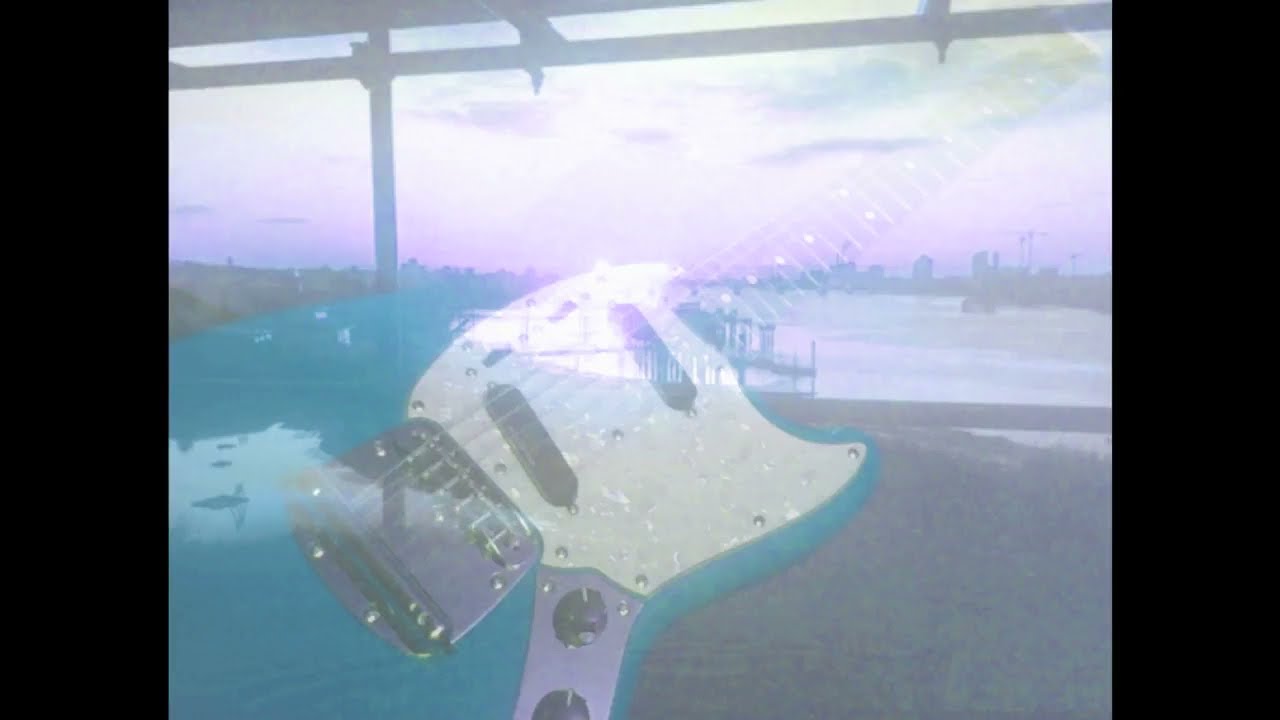The image is a layered composition featuring a distinctly visible electric guitar over a cityscape and a shoreline. The guitar, whose body is a blend of blue-green, aqua, and teal hues, has a white center panel and a shiny chrome area around the knobs, with a brown wooden neck. The guitar appears somewhat transparent, as if overlapped or blended into the background, creating a fused effect. This background showcases an industrial city view with high-rise buildings and a sprawling body of water. The scene includes a grassy area from where the picture might be taken, and it captures the sky during a daytime sunset, filled with a purple haze, patches of gray clouds, and hints of yellow and orange. The sky is further accented by a horizontal black bar at the top and two vertical black bars framing the image. Together, the elements create a soft, hazy effect, with a white layer giving the entire picture a dreamy, mist-covered appearance. This composition could likely serve as artwork for an album cover or a still from a music video.